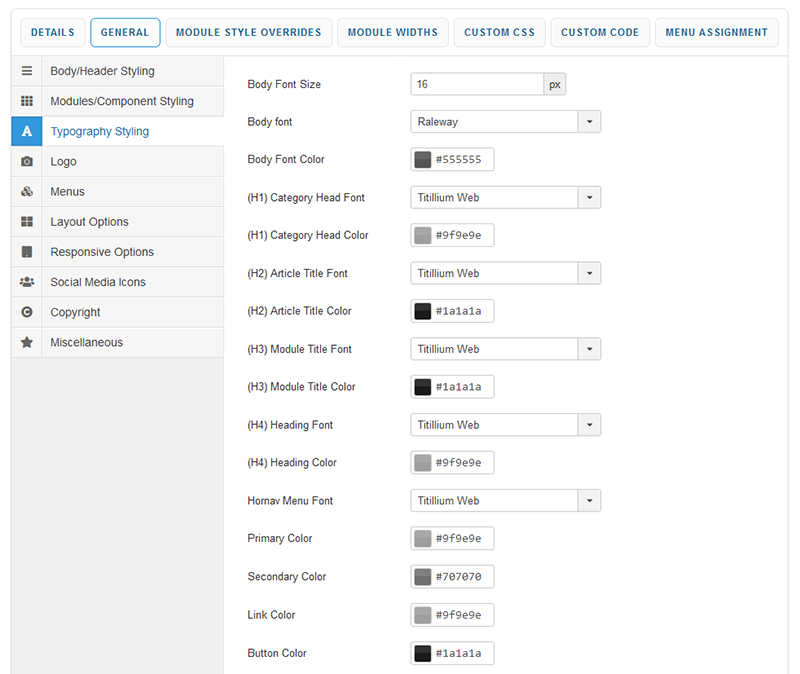The image is a detailed view of a webpage's interface, largely square in shape and outlined by a thin gray border on the top and sides, though not on the bottom, indicating the page is scrollable. The background is primarily white with a pale gray sidebar occupying the left quarter to third of the screen, featuring a vertical menu in black text. Each menu item is accompanied by a small icon. The menu options are as follows: Body Header Styling, Module/Component Styling, Typography Styling, Logo, Menus, Layout Options, Responsive Options, Social Media Icons, Copyright, and Miscellaneous.

The current selection is 'Typography Styling,' highlighted in blue with its corresponding icon enclosed in a blue box. This selection causes the main area of the page, which is white, to display various typography settings. At the top of the interface, there are seven pale gray rectangular buttons with blue capital letters, labeled from left to right: Details, General, Module Style Overrides, Module Widths, Custom CSS (Cascading Style Sheets), Custom Code, and Menu Assignment. The 'General' button is currently selected.

In the main white area on the right, there are multiple drop-down menus and input fields for configuring typography settings. These options include Body Font Size, Body Font, Body Font Color, H1 Category Head Font, H1 Category Head Color, H2 Article Title Font, along with ten other options for setting Primary and Secondary Colors, Link Colors, Button Colors, and more.